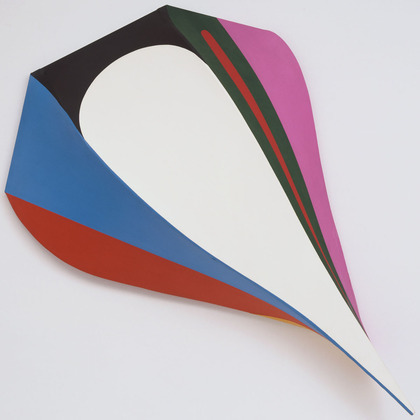The image depicts an origami-like sculpture resembling a U-shaped or C-shaped form, extending diagonally from the top left to the bottom right against a mostly white or gray background. The back of the sculpture, located at the top left, is completely black, creating a stark contrast with the rest of the piece. The right side of the shape features a predominantly black area with a red stripe running through it, transitioning into a purple outer edge and a pink, slightly curved section at the bottom. The left side displays a blue and brown composition, with blue on the inner part and brown outside. The blue section extends into the lower right area, meeting a red bottom section. The ends of the shape are pointed and thin, almost joining together at the lower right corner, suggesting a folded or layered appearance. There is a subtle shadow along the lower part adding depth, making the piece look like an abstract, multicolored sculpture or painting, possibly crafted from paper.